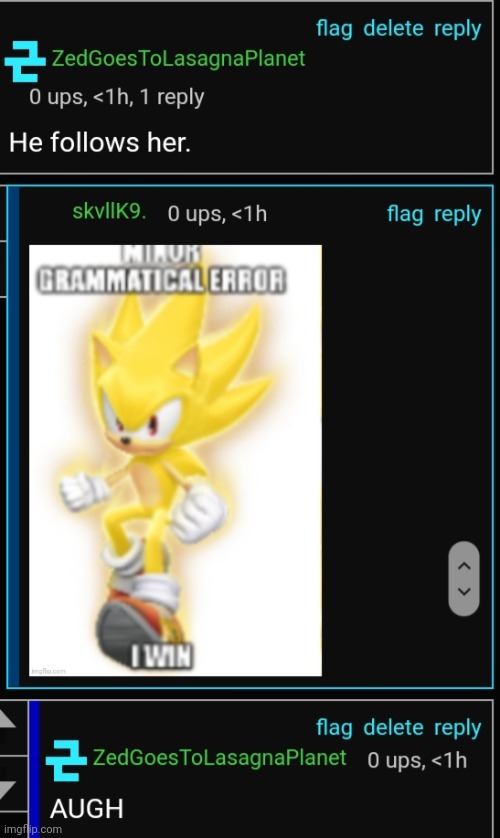The screenshot depicts a user interface, likely from a mobile game displayed on a tablet. The game interface features a black background with various elements and indicators.

In the upper left corner, there is an unusual turquoise aqua icon resembling a digital number "2" with a hyphen across the middle. To its right, in green text, it reads "Zed goes to lasagna planet" as a single concatenated word.

In the upper right corner, there are options for "flag," "delete," or "reply." Below that, the first line in the upper left corner shows "zero UPS, less than one hour, one reply." 

The main body of the screen features a series of interactions. In white text, it states, "he follows her." Below this text, there's a blue-bordered section containing a username, possibly "SKVLLK90UPS," and mentions "under one hour," along with options for "flag" and "reply."

The screen then shows a graphic on a yellow background. This graphic depicts what appears to be a cat with flaming yellow spikes or hair pointing in all directions, wearing white gloves. Above this graphic, the text reads, "minor grammatical error," and at the bottom, it states "one win," implying a gameplay or achievement element.

Overall, it looks like a minimalistic game involving two players. The game seems to focus on interactions and corrections, possibly within a narrative or text-based format.